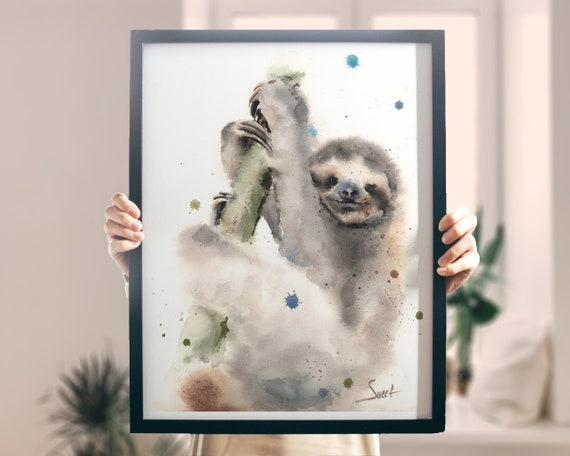The photograph captures a person, likely a woman based on the visible hands, standing in a minimally decorated room with white walls and two doors. Behind her, there are green plants adding a touch of nature to the otherwise simple setting. The person is holding up a framed painting, prominently featuring a sloth in watercolor. The artwork, enclosed in a black frame, depicts the sloth clinging to a stick or piece of bamboo. The painting is primarily black and white with deliberate splashes of blues and browns that give it an abstract, slightly unfocused appearance. The bottom right corner of the painting bears an unreadable signature that starts with an "S" and ends with a "T." The overall composition of the room is enhanced by the presence of a small window seat, partially visible with a cushion on it.